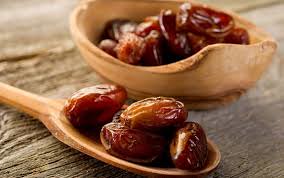A close-up image captures a rustic, unsmoothed wooden table with visible grayish-brown ridges. Resting on this table is a hand-carved, brown wooden spoon holding four date-like fruits. These fruits are reddish-brown, slightly wrinkled, with a texture that suggests softness, and you can almost see the skin peeling off. Beside the spoon is a matching wooden bowl, slightly irregular in shape with a flat edge, containing more of these dried, reddish-brown dates. The overall setting exudes a rustic charm, likely part of a recipe page showcasing the ingredient in detail.